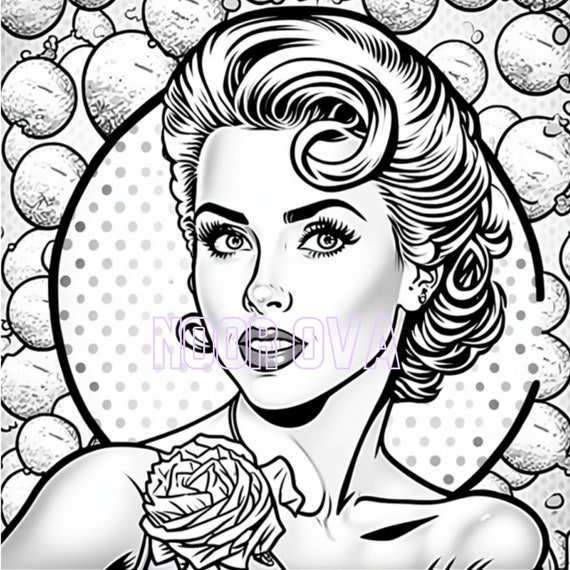This black and white pop cartoon image features a beautifully drawn woman as the central figure. She exudes elegance with her chin-length, curly hair and striking facial features, including dark eyebrows, lush eyelashes, an upturned nose, and full, darker lips. The image captures her from the shoulders up. Adorning her right shoulder is a distinct red rose. Surrounding her head is a large, dark circular backdrop filled with varying shades of polka dots, adding depth to the composition. The rich assortment of soap bubble-like shapes scattered throughout the background enhances the whimsical atmosphere of the drawing. Prominently displayed across the bottom of her face is the text "Norova" in purple outline letters, serving as both a watermark and a signature style indicative of the artist.